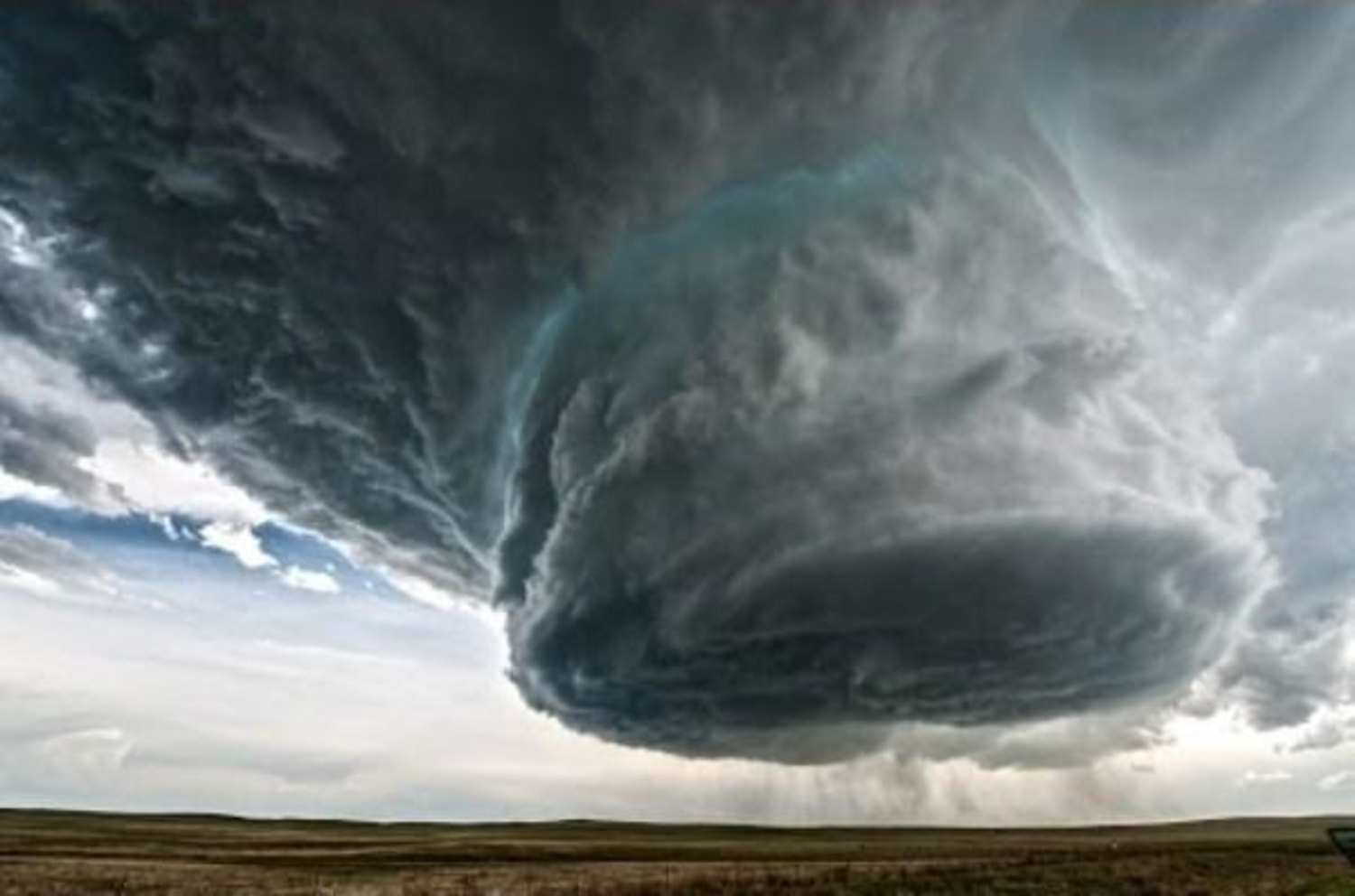This horizontally aligned rectangular image portrays a large, dramatic cloud formation against a sky with a countryside field below. The top three-quarters of the picture is dominated by this massive cloud, which begins wide and dark gray in the upper left and stretches across to the upper right. As it narrows towards the middle, it transitions into a cylindrical shape with dark gray at the bottom and intricate details of white and gray sides. Vertical streaks, possibly rain, descend in the background. A sliver of bright blue peeks through where the cloud formation narrows. Below these clouds, the bottom strip of the photo shows a field with mixed shades of green and brown, suggesting a Midwest-like open plain with no visible structures. The scene has an eerie, almost surreal quality, with the swirling motion of the clouds hinting at a tornado that appears moments away from touching down, yet not entirely realistic, potentially giving the impression of a computer-generated image.